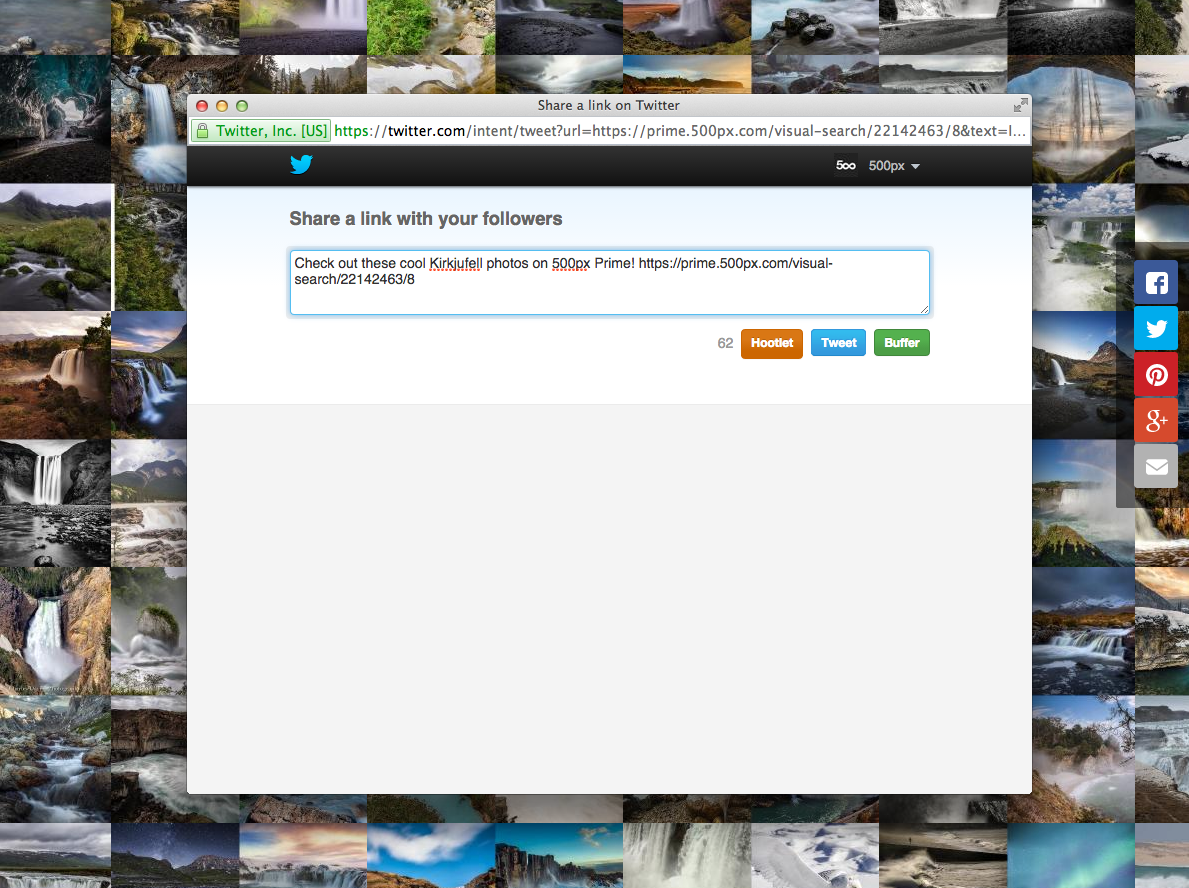The image features a computer screen displaying a website. The screen has an elongated rectangular shape typical of a computer display. The background of the screen is a collage of various waterfall images, showcasing different seasons. Some waterfalls are frozen, indicating winter, while others are flowing, representing summertime.

Superimposed on this background is a white and gray rectangular window that appears to be an open Twitter share dialog. The URL in the address bar reads "twitter.com/intent" followed by a series of numbers and words, indicating a link-sharing page. The text within the dialog box prompts the user to "share a link with your followers," with the main message stating, "Check out these cool Kirk Jufel photos on 500px Prime," followed by a clickable HTTPS link.

Below this text, there are three interactable buttons: 
1. The first button, labeled "Hootlet," has an orange background with white text.
2. The second button is blue with the word "Tweet" in white text.
3. The third button, green with the word "Buffer" in white text, is the final option on the dialog box.

The detailed composition of the screen suggests a focus on social media engagement and content sharing, set against a visually rich background of seasonal waterfalls.